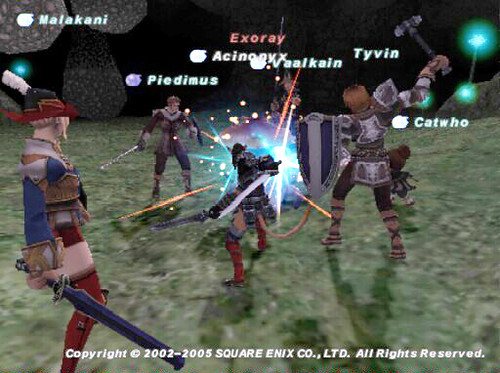This color screenshot from a video game captures an intense battle scene with four players. Dominating the left center bottom of the image, a man stands vertically wielding a sword, attentively observing the action unfolding. In the center, combatants equipped with shields and swords are locked in fierce confrontation, some clutching various objects. The pixelated scene is electrified by a brilliant explosion of blue light, accented with sparks and vivid orange lines radiating from the epicenter of the clash. Player labels are displayed along the top part of the image, providing context for the action. At the bottom, white text states, "Copyright 2002 to 2005, Square Enix CO, limited, all rights reserved." The entire scene, slightly pixelated, features bright yet muted and pale colors, evoking a retro yet dynamic visual aesthetic.